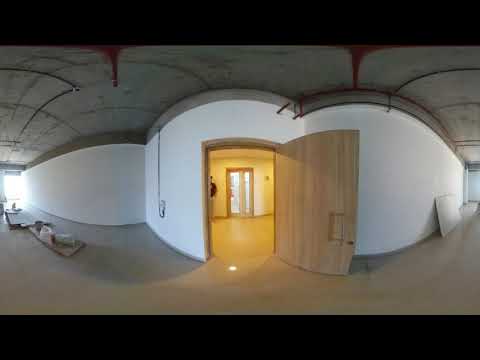The image showcases the entrance of a modern building, potentially a commercial or under-construction space. The interior walls are white, complimented by an exposed concrete ceiling and grayish flooring. Centrally placed in the composition is a prominent, light wood door with a pole handle, which stands open. This door leads into a well-lit hallway with a shiny, possibly tiled floor illuminated by yellow lighting. Across this hallway is another door, featuring a glass panel, which is currently closed. A partially visible person appears to be leaning against the wall next to this interior door, offering a glimpse of human presence. The scene also details various items scattered on the floor to the left of the main door, reminiscent of construction materials, including boards and possibly paint buckets. Additionally, emergency water pipes are visible on the right side of the image, contributing to the industrial and unfinished ambiance of the space.